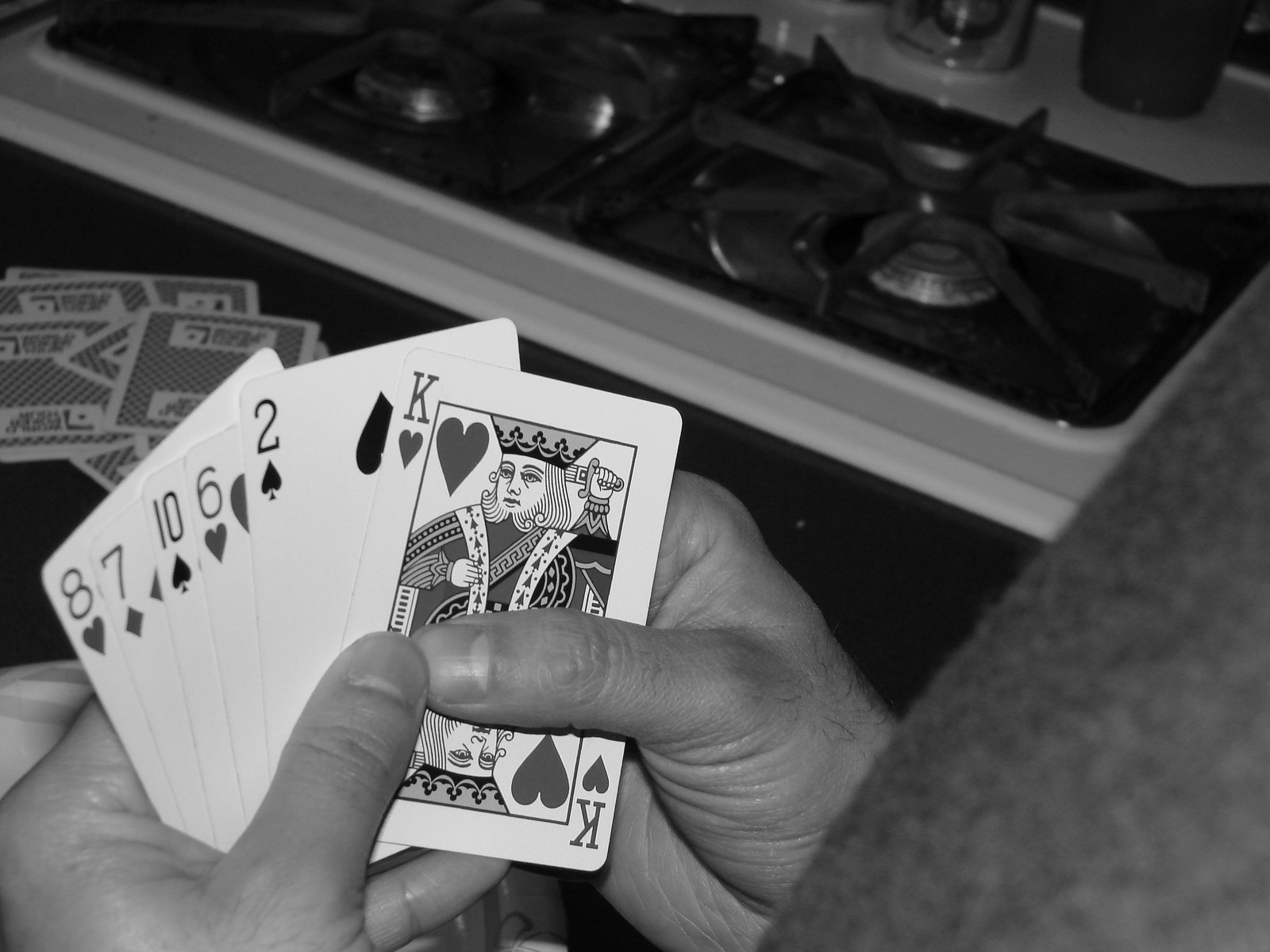In this evocative black and white photograph, the viewer is given an intimate over-the-shoulder perspective of an individual engrossed in a card game. Their hands, central to the composition, crisply display a neat spread of cards, with their sequence reading from left to right: the eight of hearts, seven of diamonds, ten of spades, six of hearts, two of spades, and king of hearts. The careful arrangement of the cards suggests the person is in the midst of organizing their hand for an unknown card game. The tableau is set on a modest table, scattered with a few other cards, hinting at the ongoing nature of the game. Surrounding them, the backdrop is a quaint kitchen scene, centered around a small, utilitarian stove typical of an extended-stay hotel or cozy studio apartment. The stove, situated in the upper part of the photograph, features two black burners contrasted against a white surface with black edges, blending perfectly with the monochromatic palette. The player wears a dark-colored shirt, but the grayscale effect leaves the precise hue to the imagination. Overall, the image captures a fleeting, quiet moment of focus and strategy in a small, humble setting.